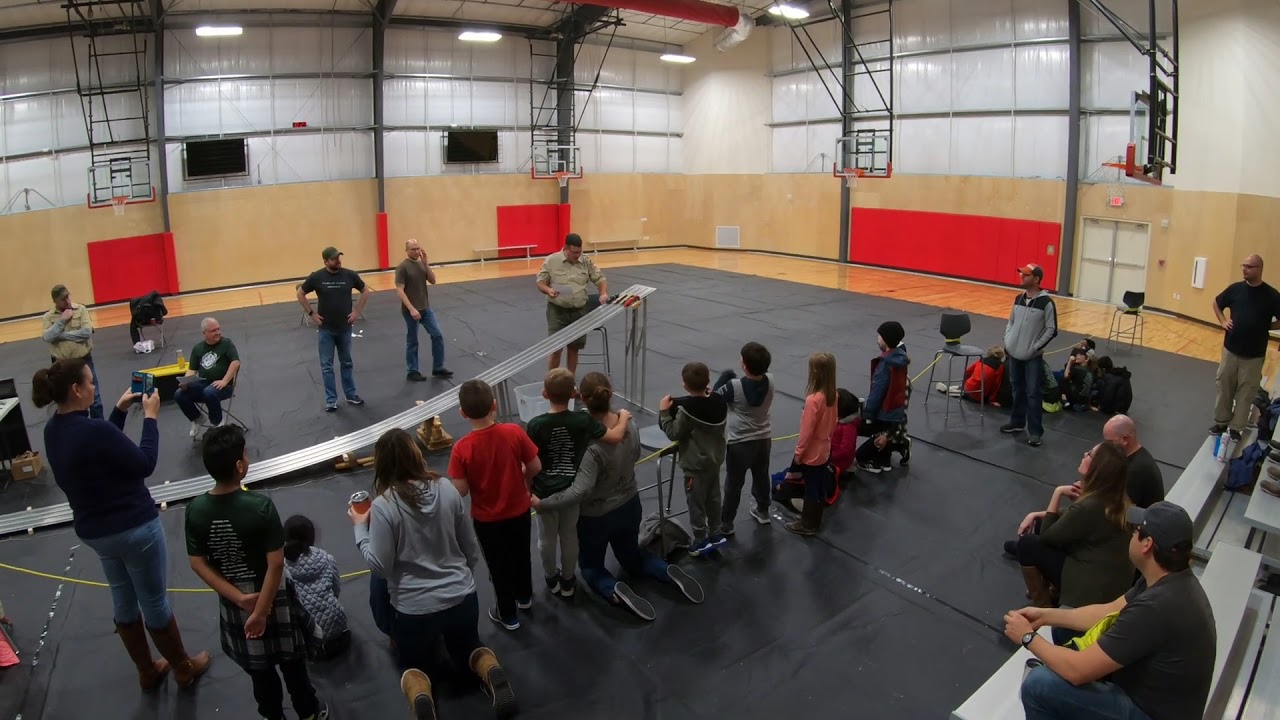In a bustling gymnasium, a focal point is the Pinewood Derby race setup, where multiple people, including young children and adults, are keenly observing a scout leader in a tan button-up shirt and green shorts. He carefully places model-sized vehicles onto a sleek, silver ramp positioned at the center of the scene, preparing them for the race. To the right, several spectators are seated on silver-colored bleachers, intently watching the event unfold. The floor is predominantly covered by a black gym mat, with light-colored wooden sections peeking through along the perimeter. On the left, a woman records the proceedings with her phone. The gym's walls feature occasional red mats and are adorned with multiple basketball hoops suspended from the ceiling. Brightly illuminated, the gym is a lively setting for the community gathered to witness the excitement of the Pinewood Derby race.